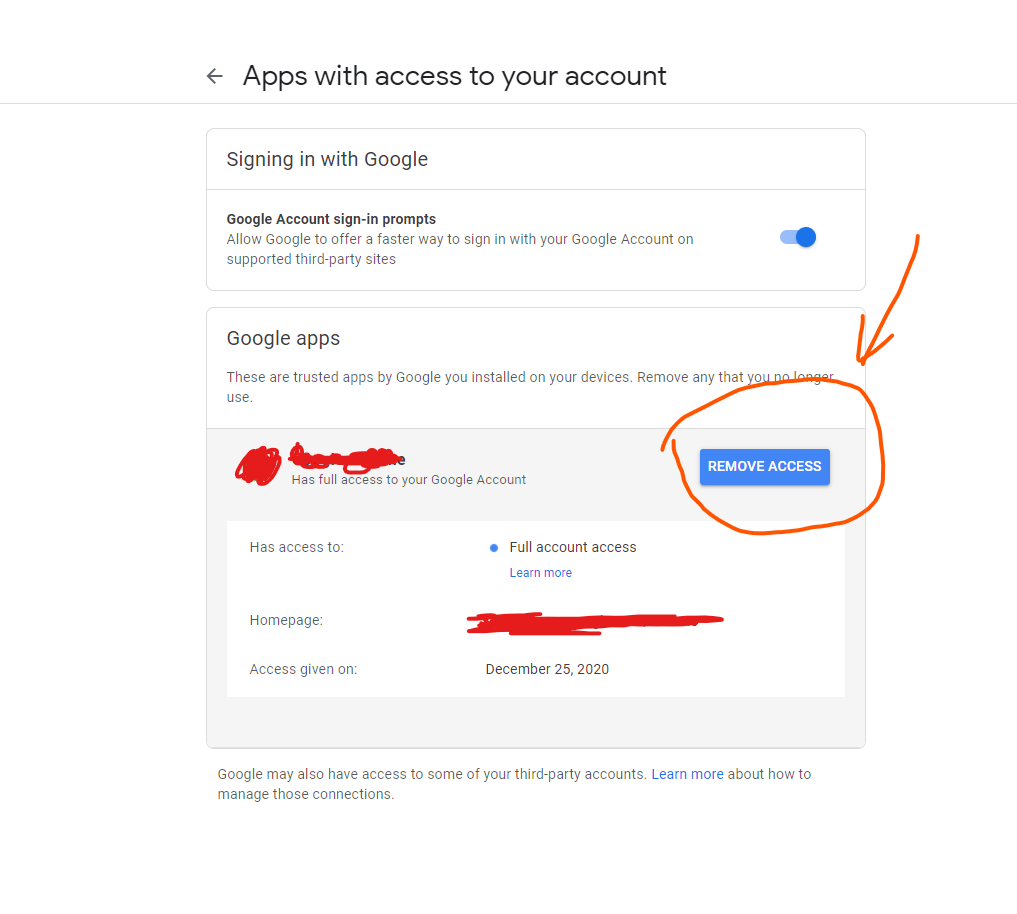A detailed screenshot of a Google account settings page: At the top, the page header reads "Apps with access to your account," preceded by a left-facing arrow. Below this header, a white section labeled "Signing in with Google" is visible, followed by another white section stating "Google account sign-in prompts." This section includes a brief description: "Allow Google to offer a faster way to sign in, sign in with your Google account on supported third-party sites," with a toggle switch set to "on" on the right side.

An arrow, drawn on the screenshot, directs attention to the middle section titled "Google apps." This section notes that these are trusted apps installed on your devices and advises to "Remove any that you no longer trust." At the bottom of this section, a gray area contains some obfuscated text, except for the phrase "has full access to your Google account." Adjacent to this, a circled "Remove access" button is highlighted by the previously mentioned arrow.

Further down, another white section reads "has access to," accompanied by a blue button marked "full access." Below this button is a "Learn more" link. The section continues with details, including a gray box with red scribbles obscuring the text, except for the phrase "access given, December 25th, 2020." The final note outside the gray box mentions, "Google may also have access to some of your third-party accounts," with an additional "Learn more" link providing information on managing those connections.